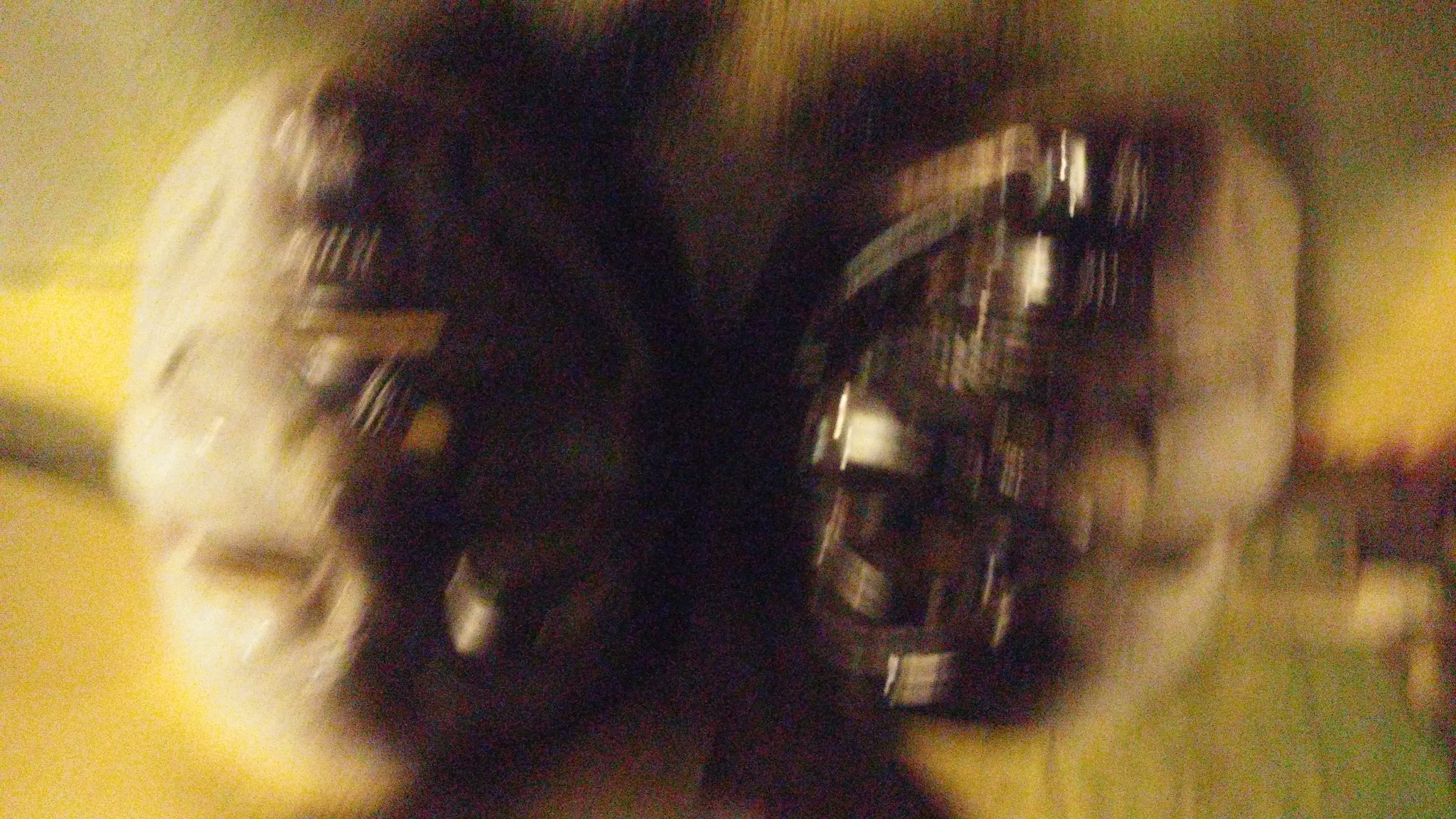In this image, the foreground features two slightly blurred objects on a table, which appear to be masks. The masks are presented in different orientations: the mask on the left is upside down, revealing two eyes near the bottom along with a vague outline of a nose and mouth, rendering its facial features faint. The mask on the right, in contrast, is right side up and more detailed, distinguished by an intricate braided pattern running horizontally across the left side. The combination of these elements creates a sense of artistic complexity and adds a mysterious atmosphere to the image.